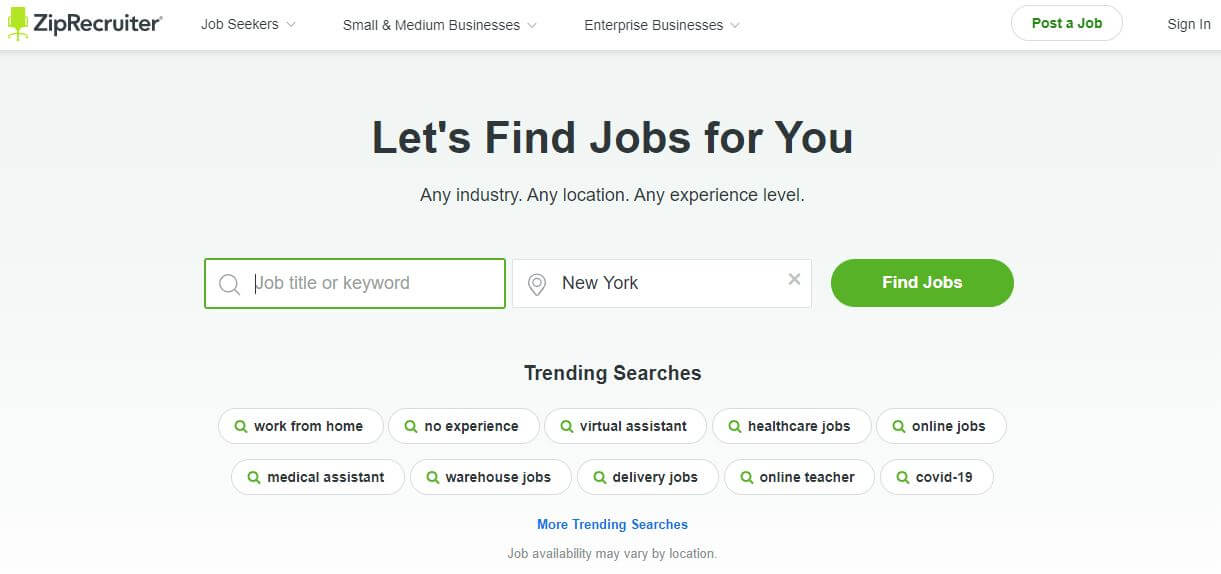The image depicts the homepage of the ZipRecruiter website. In the top-left corner, there is an illustration of a lime green office chair. The name "ZipRecruiter" is prominently displayed in bold black letters. 

At the top of the website, there are navigation categories labeled "Job Seekers," "Small & Medium Businesses," and "Enterprise Businesses." On the right side of the navigation bar, there is a green button with gray outline and a white circle that reads "Post a Job." Adjacent to it is a "Sign In" link.

Below the navigation bar, within a light gray box, a welcoming message encourages users to find jobs with the text: "Let's find jobs for you. Any industry, any location, any experience level." Beneath this message, there is a search bar where users can enter a job title or keyword. The specified location is "New York," and a green button labeled "Find Jobs" in white text is located next to the search bar.

Further down, there is a section titled "Trending Searches" in black text, which lists popular job categories such as "Work From Home," "No Experience," "Virtual Assistant," "Health Care Jobs," "Online Jobs," "Medical Assistant," "Warehouse Jobs," "Delivery Jobs," "Online Teacher," and "COVID-19." Additionally, there is a blue link labeled "More Trending Searches" with a note underneath in black that reads, "Job availability may vary by location."